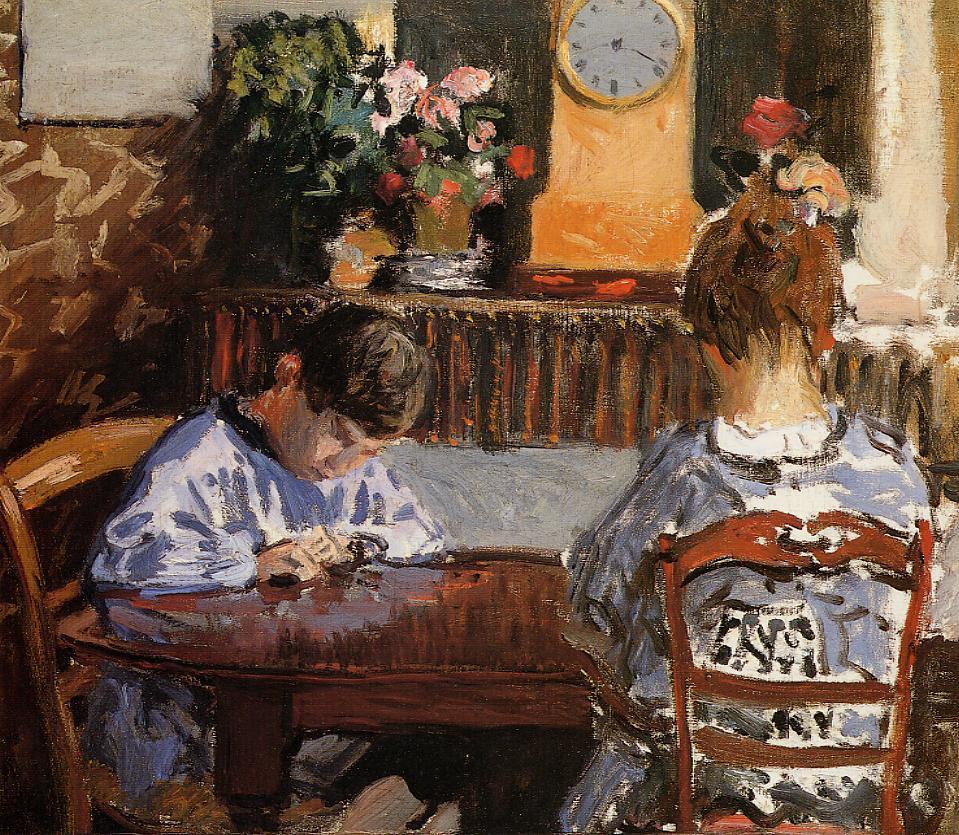This detailed oil painting captures an intimate scene set in what appears to be a dining room. At the bottom of the image, a dark brown, glossy table serves as the central focus. A young girl with light brown hair styled in a ponytail sits with her back to the viewer in a dark brown, intricately designed chair on the right side of the table. She is dressed in light blue and black. Across from her, a young boy with dark brown hair, also dressed in light blue and black, looks down at the table with both fists placed firmly on it, perhaps engaged in an activity. He sits in a light brown wooden chair. Behind them, a fireplace adorned with a tall, golden clock and a modest arrangement of flowers creates a warm ambiance. The background wall is an elegant mix of black bordered in white, adjacent to a brown wall with a window, contrasting subtly against the gold-toned wall on the right. The high-definition presentation of this painterly artwork accentuates the details, making them vivid and lifelike.